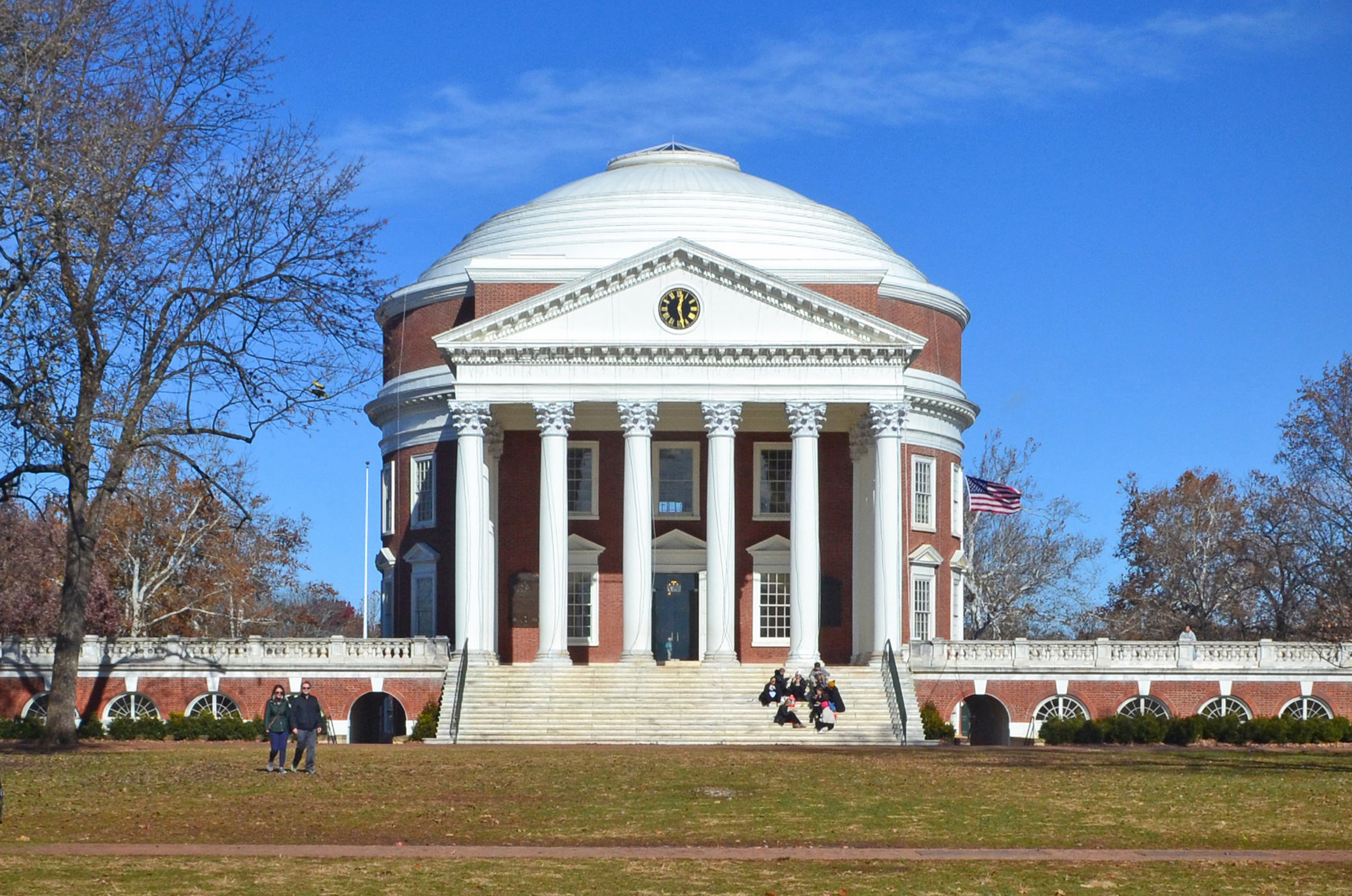The photograph captures a historical building that evokes the architectural style of several hundred years ago. The structure, which is reminiscent of Monticello but likely not, is situated in an outdoor setting with a clear view of the large, white, rounded dome at the top. The front of the building features six narrow columns that support a triangular pediment. Above the columns, there's an embedded black and gold clock. The building is constructed from brown-red brick with white trim around its multiple windows, indicating it has at least two stories. 

An expansive set of white steps, flanked by a red brick wall and white railing, leads up to the entrance. To the right of the building, from the viewer's perspective, an American flag is prominently displayed. The scene is set against a backdrop of mostly bare trees, suggesting the photo was taken in the fall. On the steps, a group of four to five people can be seen, though their attire is indistinct. Additionally, two individuals are walking on the green lawn in front of the building, one in a green jacket and the other in a dark blue jacket, both wearing jeans or dark trousers. The building exudes an official, stately vibe, possibly indicating it serves an important public or governmental function.